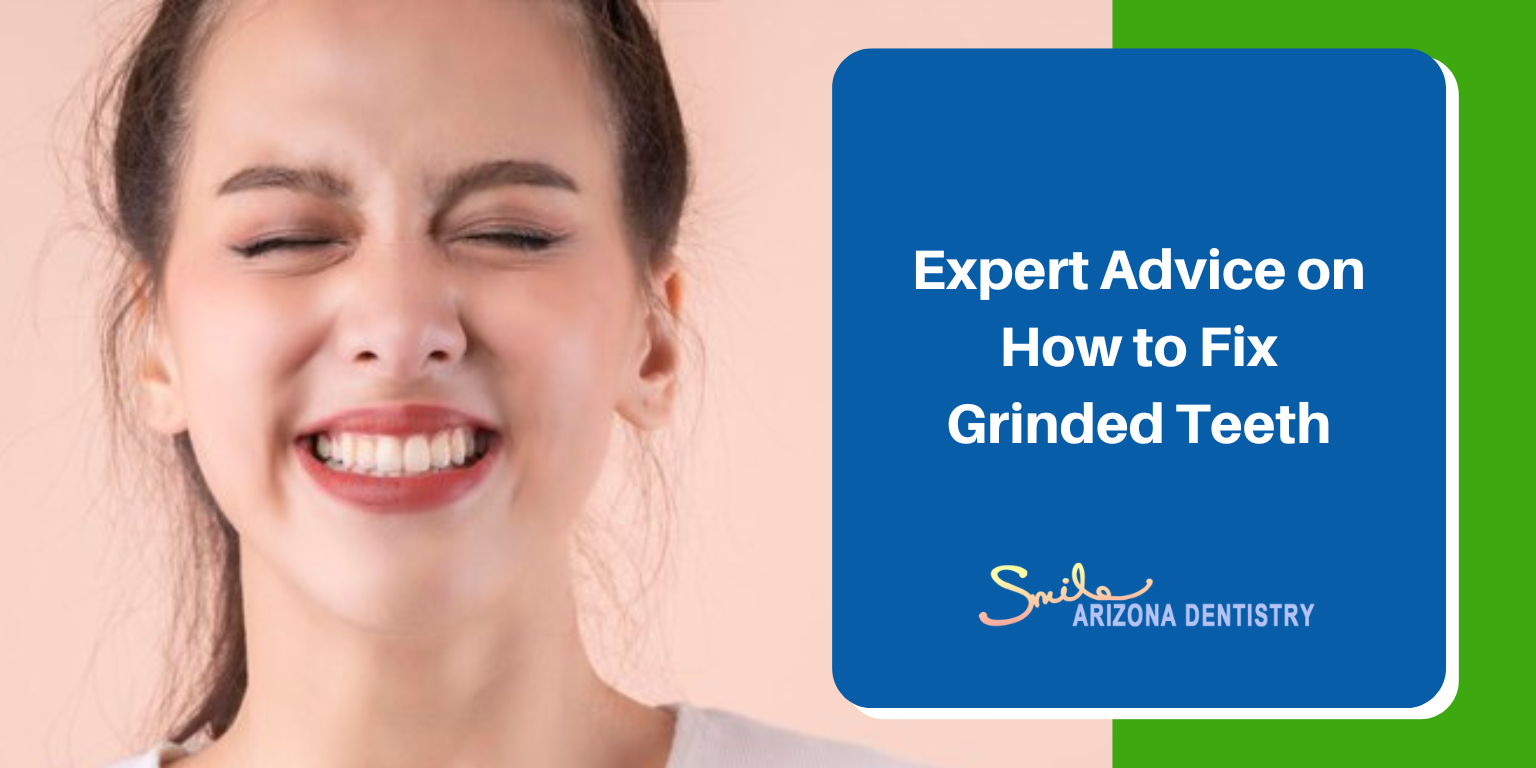The digital advertisement is a wide rectangular image predominantly featuring a photograph of a woman on the left-hand side and text on the right. The woman, with pale yet slightly warmer skin than the background, has her eyes closed and is giving a broad, toothy smile that reveals her teeth. She has brown hair styled in an updo and brown eyebrows. Her eyelids are adorned with bronze eyeshadow, and her thick lips are coated with red gloss.

To the right of her face, there is a blue square with curved corners, containing the white text "Expert advice on how to fix grinded teeth." Below this in cursive yellow, it says "Smile." Further down, in gray text, it reads "Arizona Dentistry." The far right edge of the advertisement features a green background, adding a contrasting pop of color to the design. The overall image is designed to highlight the dental services offered by Smile Arizona Dentistry, focusing on solutions for teeth grinding, as indicated by the accompanying text and the woman's highlighted smile.